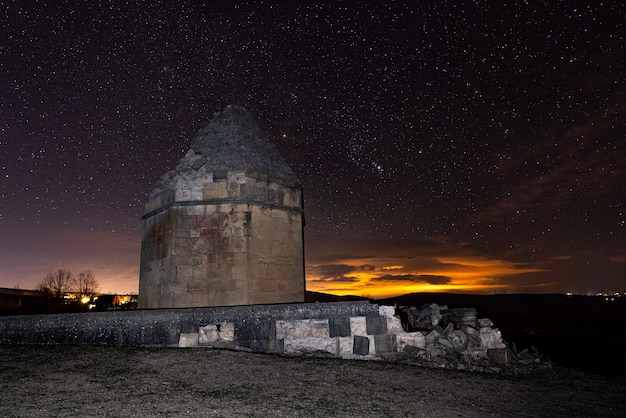The photograph captures a hauntingly beautiful scene set at twilight in a desolate, open field. At the center stands an abandoned, bullet-shaped building, possibly a silo, weathered and crumbling with time. The lower part of the building is a brownish hue, marred by dark stains, while the upper part is charred black, likely from a past fire. The structure sits on a deteriorating concrete or rock platform, surrounded by a low wall. The dilapidation of the building contrasts starkly with the serene landscape. Behind the ruin, the night sky is resplendent with stars, illuminated by the faint glow of a setting or rising sun, casting an orange band of light along the horizon. The scene feels remote and isolated, with only a few distant trees casting shadows in the background, emphasizing the solitude and timelessness of this forgotten place.